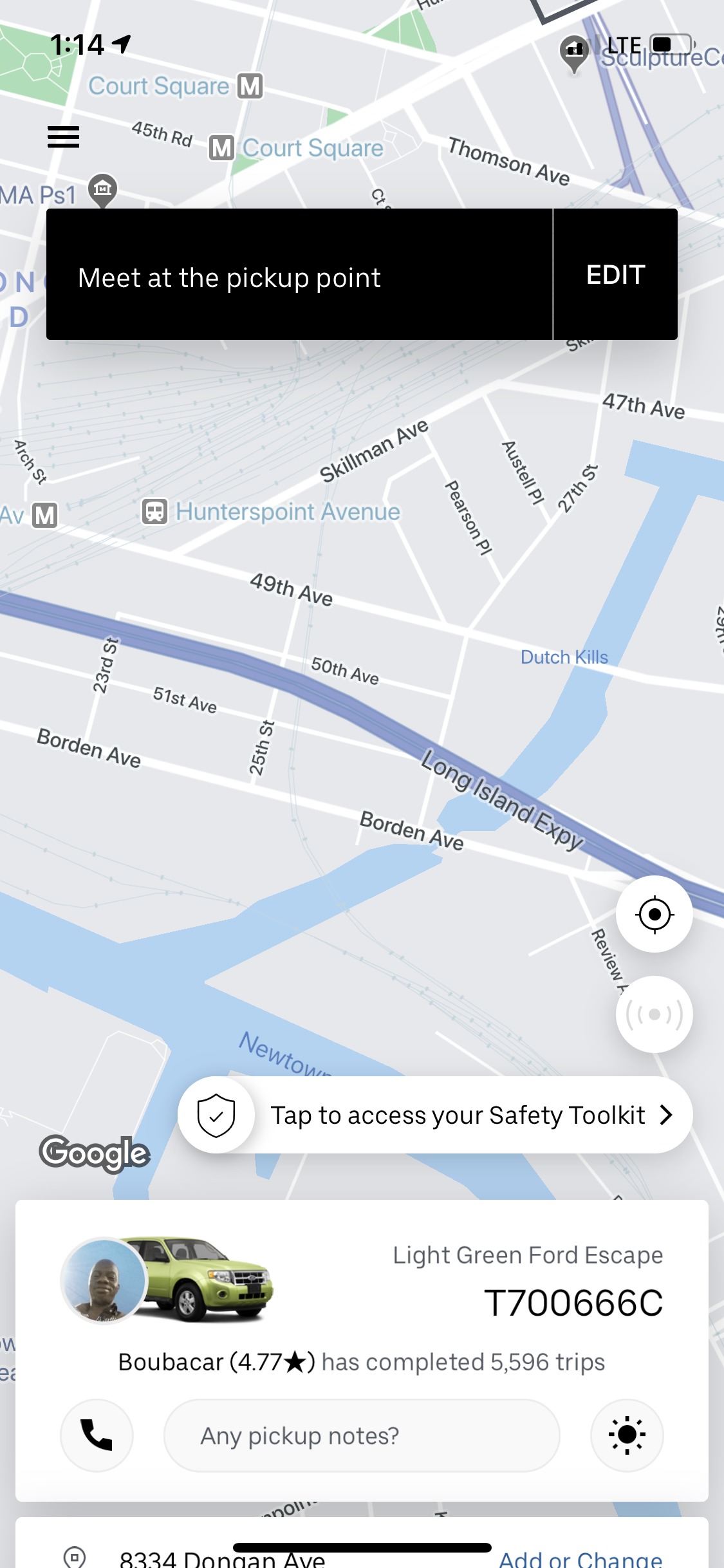This image is a detailed screenshot of a smartphone screen showcasing an Uber app interface. In the top right corner, there is an LTE signal indicator and a battery symbol, while the top left corner displays the current time and a location arrow pointing upwards. The central part of the screenshot features a map with various streets and a river visible. Across the top, a black bar contains the instruction "Meet at pickup point." Towards the bottom of the image, there is an icon of a car in white. Below this, additional Uber-specific details are visible, including a circular profile picture of the driver, the type of car they are driving, and their rating. This organized layout and specific elements confirm that the screenshot is from the Uber app, providing users with real-time and user-specific information for their ride.